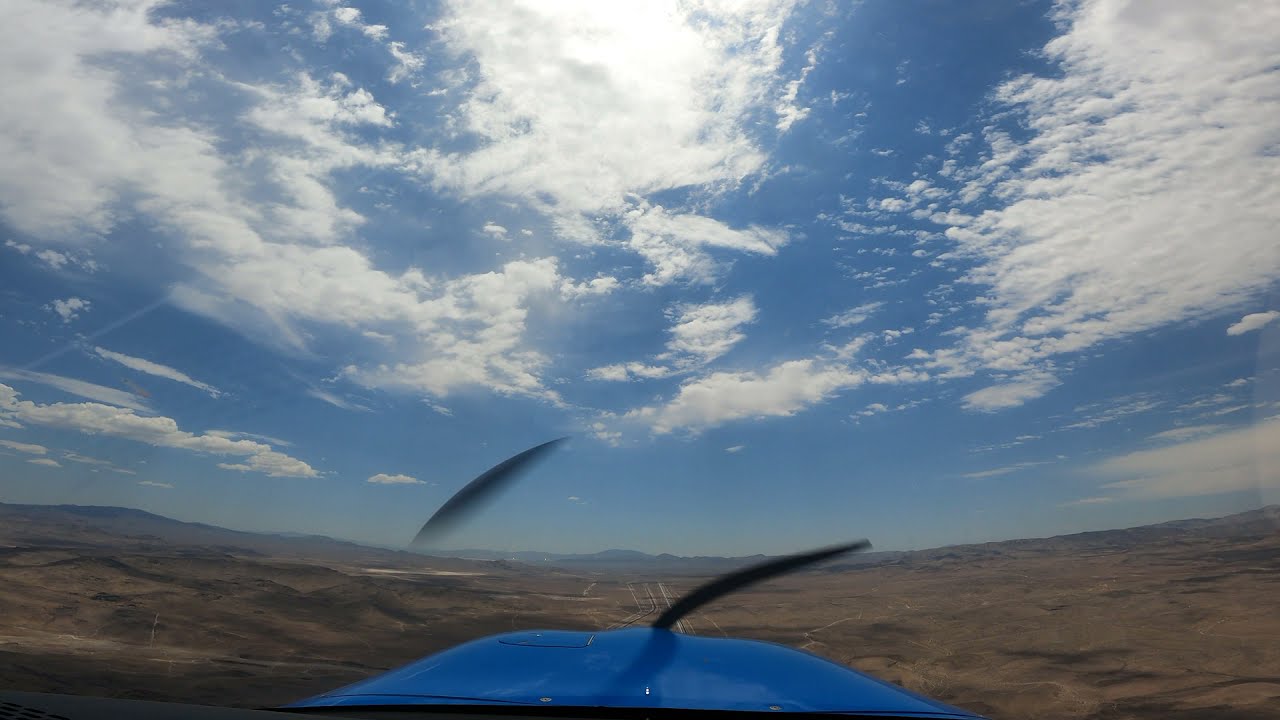The image appears to be taken from the cockpit of a small airplane flying over a barren, desert-like terrain. The propeller, caught mid-motion, creates a distorted arc in front of the camera. From this aerial perspective, the nose of the plane, painted blue, is clearly visible. The sky, occupying about two-thirds of the frame, is a lively blue adorned with scattered, thin, white clouds. Positioned prominently in the center above the horizon, the sun subtly illuminates the expansive landscape below. The ground beneath is predominantly brown, interspersed with light green streaks indicating sparse vegetation. Off in the distance, a rocky and arid mountain range stretches across the horizon, anchoring the boundary between the earth and sky. The overall scene suggests a flight over a southwestern US state like Arizona or Nevada.